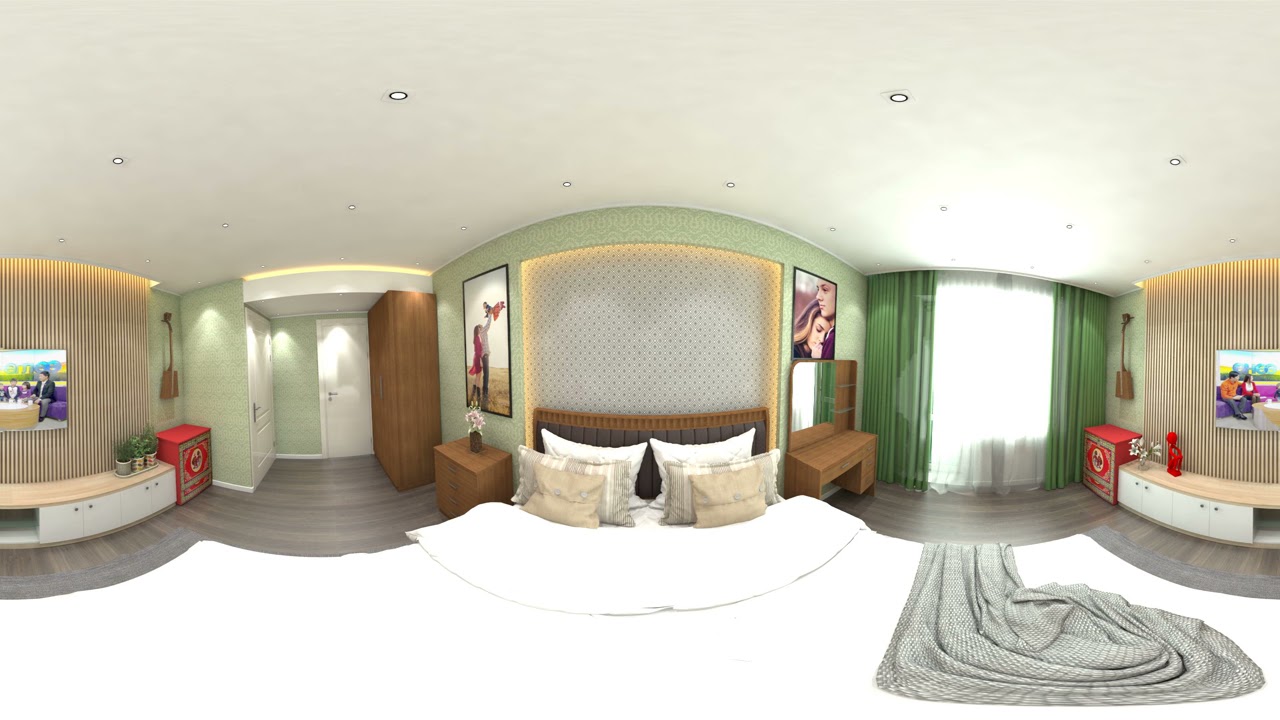The photo captures a green-walled bedroom from a slightly distorted, panoramic perspective, making the room appear curved. At the center of the image is a large, white bed adorned with six pillows: two white, two striped gray, and two beige. The bed, topped with a thin gray blanket, seems to expand outward due to the camera's distortion. A black wooden headboard frames the bed. On either side of the bed, there are wooden nightstands; one has a mirror and the other a small flower.

To the left, the furniture includes a brown dresser and a large wooden chest positioned near two doorways. Above this area, a poster featuring a person with two children hangs on the wall, accompanied by various decorations and shelves.

On the right, a poster is displayed above a desk and mirror setup, leading to a large window draped with green and white curtains. The walls and gray flooring exhibit the room's warped appearance, segmented into five sections. The white ceiling houses recessed lighting, with a couple of additional specks creating a textured look. Despite the warped view, the bedroom appears cozy and well-decorated, featuring a TV playing a show on the far side, completing the serene atmosphere.